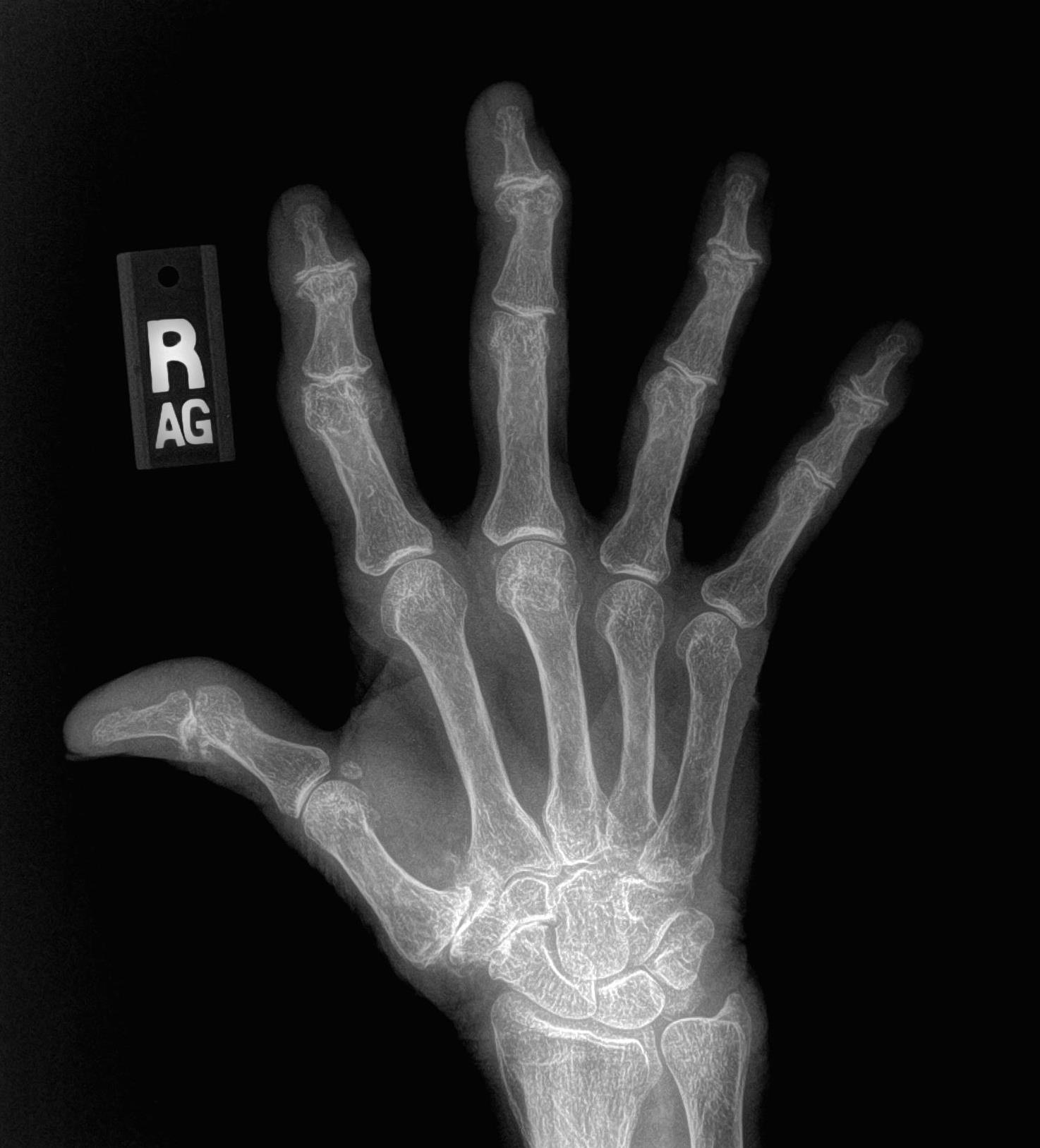This image displays an X-ray of a human hand set against a black background. The hand is positioned with the fingers slightly fanned out, and the thumb bent slightly backwards. The bones of the fingers and the hand appear white against the dark backdrop, whereas the surrounding flesh shows up as a lighter gray. Particularly, the index and middle fingers seem crooked or possibly damaged. The X-ray reveals clear details of the bones extending from the fingers into the palm and the wrist. There is also a black rectangle located in the upper left corner between the thumb and index finger that features a white letter "R" with "AG" inscribed beneath it, although one mention suggests it might be "RT". Additionally, a small device for size comparison of the hand is visible next to it.